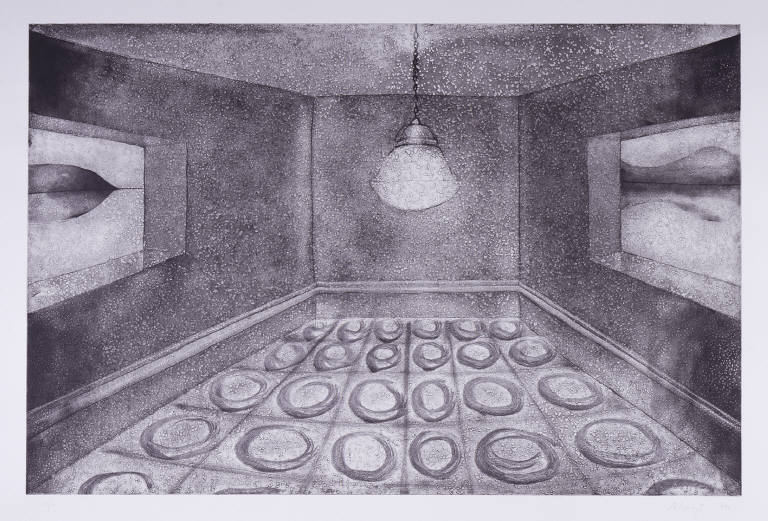This monochrome drawing, rendered in shades of gray, black, and white, depicts a stark, empty room illuminated by a large chandelier hanging from the ceiling. The detailed etching, possibly done in pencil or charcoal, reveals a futuristic and modern interior. The floor is designed in a grid pattern with each square featuring donut-shaped or oval splotches. The room's architecture includes three plain walls, with the left wall displaying a painting of a woman's lips and the right wall featuring an image of a mountain landscape, potentially hinting at a lake in the foreground. The ceiling is a somber gray, contributing to the overall muted and dark ambiance of the scene. The artwork utilizes intricate shading and white dots to create depth, giving the viewer a sense of looking into a strange, intriguing space.